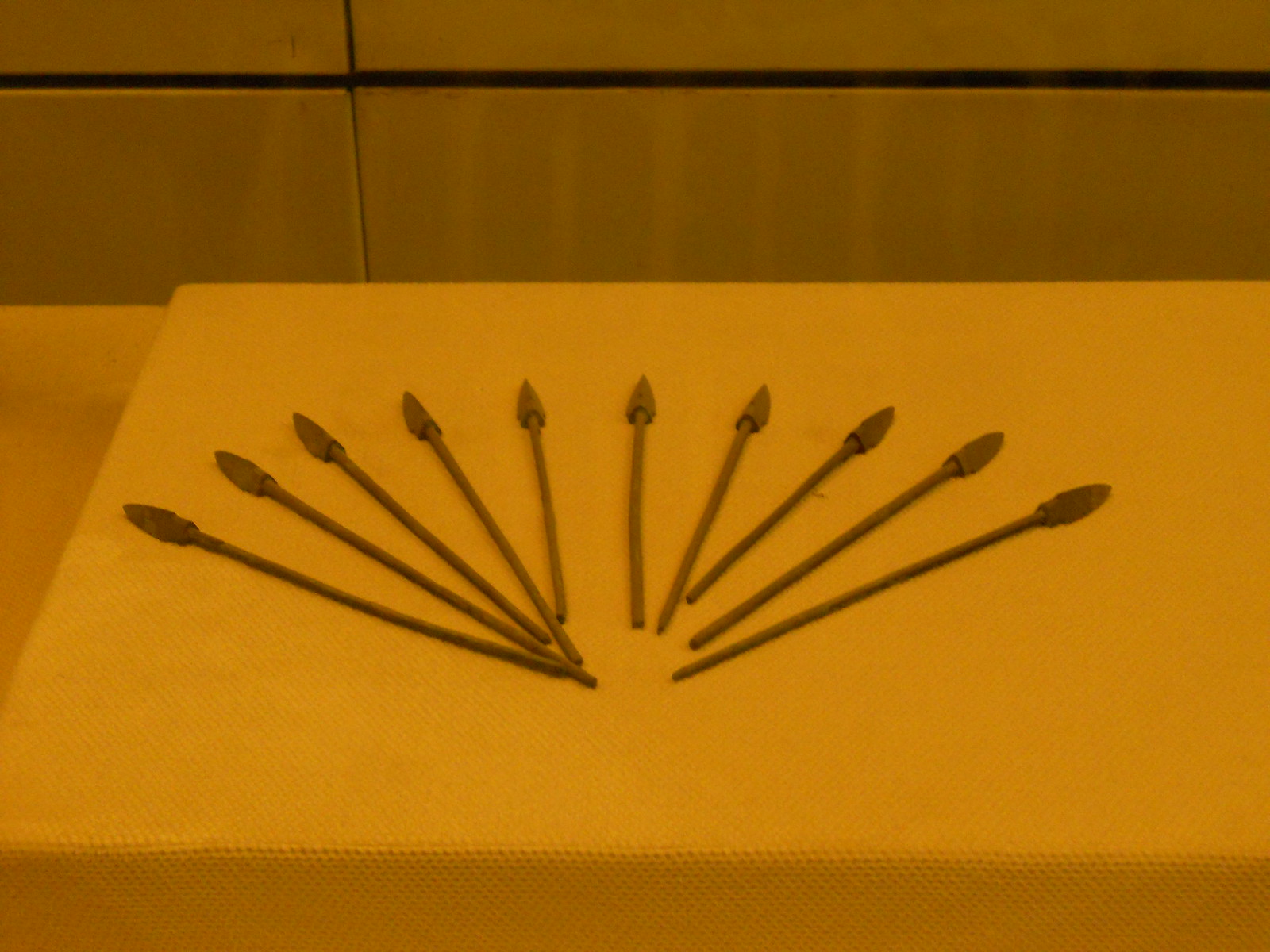This indoor photo, possibly taken in a museum, showcases a meticulously arranged display of historic wooden arrows. The arrows, with pointy spearheads, are fanned out in a peacock feather-like formation, creating a visually striking and orderly spread. There are ten arrows in total, with the two on the ends being the longest. The arrows rest on a table covered in yellow fabric with a waffled texture, imparting a warm tungsten hue to the image. The arrow shafts are a lighter brown shade, suggesting a wooden material. Behind the display, there is a brown wall comprised of panels with black gaps in between, adding depth to the background and highlighting the historic nature of the exhibit.